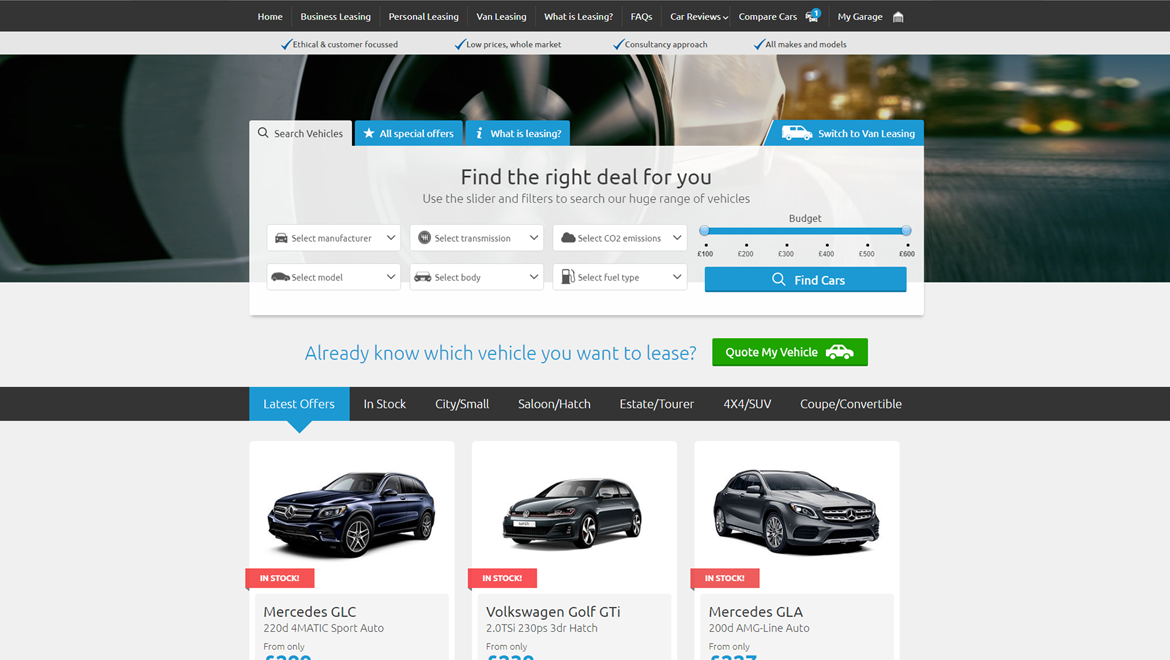The screenshot depicts a detailed interface of a rental car website.

At the top, the title bar is shaded in black or grayish color, containing several menu buttons. From left to right, the buttons are: "Home," "Business Leasing," "Personal Leasing," "Van Leasing," "What is Trending," "FAQs," "Car Reviews," "Compact Cars," and "My Garage" which features an icon. Below this bar, there is a gap containing a list of company values: "Ethical and Customer Focus," "Low Prices," "Whole Market," "Consultancy Approach," and "All Makes and Models." Each of these values is accompanied by a check mark.

Beneath this section is an image showing the right side of a car with a spinning wheel, set against a city skyline in the background.

Further down, a series of search options are presented: "Search Vehicles," "All Special Offers," "What is Leasing," and "Switch to Van Leasing." Alongside these, the slogan "Find the right deal for you" is displayed, accompanied by various search boxes to input preferences, including a budget slider.

At the bottom section, there is a "Find Cars" button followed by categories like "Latest Offers in Stock," "City Small," "Saloon," "Hatch," "Estate," "Tour," "4x4 SUV," and "Coupe Convertible." Below these categories, images representing selected or searched-for vehicles are displayed.